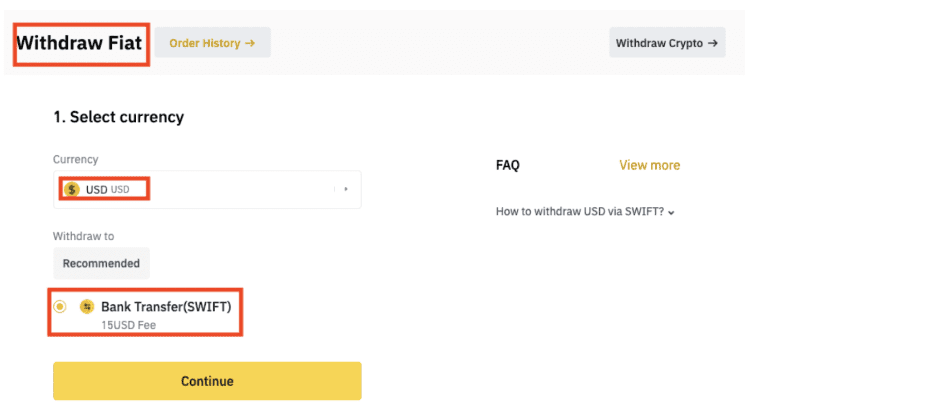**Image Description:**

This landscape-oriented screenshot features a well-organized layout with clearly defined sections, all displaying predominantly gray and white backgrounds. 

1. **Top Row:**
   - The upper left section, encased in a red-bordered rectangle, prominently displays "Withdraw Fiat" in bold black text against a very light gray background.
   - To its right, a gray button labeled "Order History" in orange text with an accompanying orange arrow is present.
   - At the far right end, a gray button labeled "Withdraw Crypto" in black bold text with a black arrow points the way.

2. **Middle Section:**
   - Below the top row, two columns with white backgrounds are displayed.
   - In the upper left-hand corner of the first column, the bold text "Select Currency" is visible.
   - Following it is a form section starting with the label "Currency" in gray text adorned with an asterisk indicating a mandatory field.
   - An icon featuring a gold circle and black 'US dollar' symbol appears next to the text "USD" in both bold black and gray text. This section is surrounded by a defining red rectangle.
   - The next part of the form reads "Withdraw To" in gray text, followed by a gray button labeled "Recommended" in dark black text.
   - Directly below this, enclosed within another distinct red rectangle, is the "Bank Transfer (SWIFT)" option.
   - An orange button labeled "Continue" stands at the bottom of the column, signifying the next step in the process.

The screenshot demonstrates a clean and user-friendly interface, with essential buttons and options organized efficiently for ease of access.